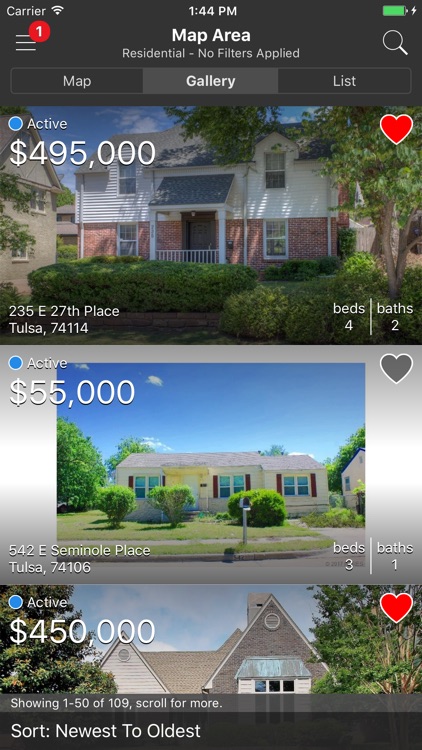The image captured from a smartphone screen displays a real estate app interface featuring three property listings for sale. At the top of the screen, a header reads "Map Area - Residential, No Filters Applied" in white text against a black background. To the right of this header is a search button, while on the left is a menu button displaying a red notification badge marked with the number one.

Below the header, there are three navigational tabs labeled "Maps," "Gallery," and "List." The "Gallery" tab is currently selected, showcasing three houses. 

The first listing in the gallery is an active property marked by a blue dot on the left side. The house is priced at $495,000, indicated in white text, and located at 235 E 27th Place, Tulsa, 74114. It features four bedrooms and two bathrooms. A red heart icon on the top-right corner indicates that this property is liked.

The second listing, also active with a blue dot, is priced at $55,000. It is located at 542 E Seminole Place, Tulsa, 74106, and offers three bedrooms and one bathroom. This property has not been liked, as shown by the grey heart icon on the top-right corner.

The third listing is another active property priced at $450,000, with a red heart icon indicating that it is liked. The property's detailed location and features are not expressly reiterated in the description, but it implies the presence of a similar layout as the other listings.

At the bottom of the screen, the sorting criterion is displayed as "Sold - Newest to Oldest."